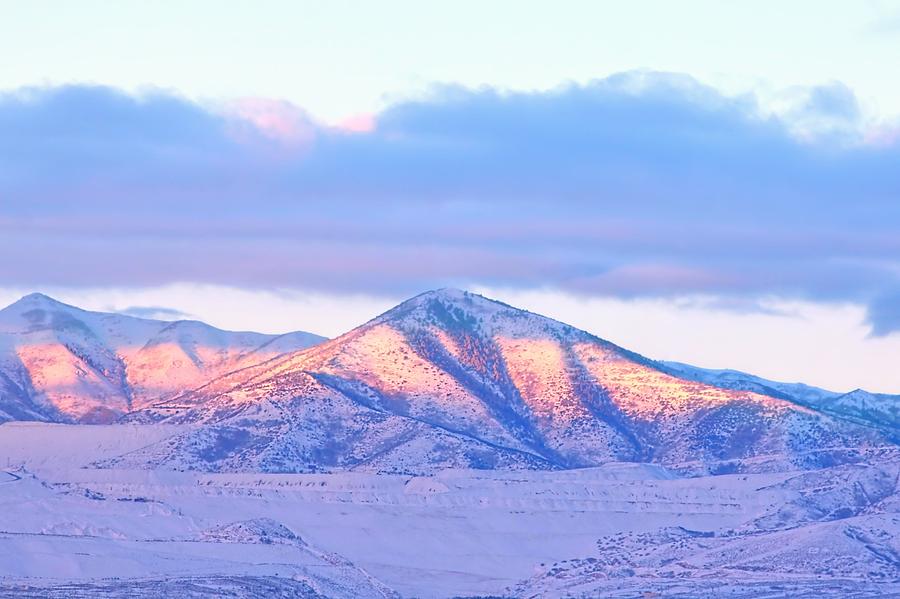This photograph captures a spectacular mountain range blanketed in snow. The central peak, shaped more like a hill than a rocky summit, is bathed in a band of sunlight that casts a striking orange and yellow glow across its snowy surface, creating the illusion of lava-like reflections. Above, a mix of light and dark blue clouds stretch horizontally, partially shrouding the mountaintops while leaving patches of sky visible. The foreground shows a gently snow-covered valley, with ridges and sunken valleys nestled between the peaks. Overall, the sunlight piercing through the dark, shadowy expanse of snow-covered mountains creates a dramatic contrast, highlighting the unique and serene beauty of the landscape.